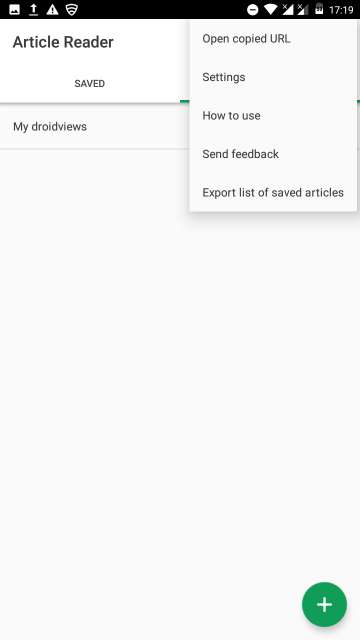Screenshot of the 'Article Reader' page from My Droid Views application. The interface features a dense black header with multiple small icons at the top, showcasing various functionalities. Below the header, the title 'Article Reader' is prominently displayed in large, bold text. A couple of lines beneath that, the word 'Saved' appears in a smaller font size, followed by the caption 'My Droid Views.' On the right-hand side of the page, there is a menu listing options including 'Open Copied URL,' 'Settings,' 'How to Use,' 'Send Feedback,' and 'Export List of Saved Articles.' The layout suggests a user-friendly environment designed for saving and managing articles within the app, allowing users to easily access and organize their reading material.